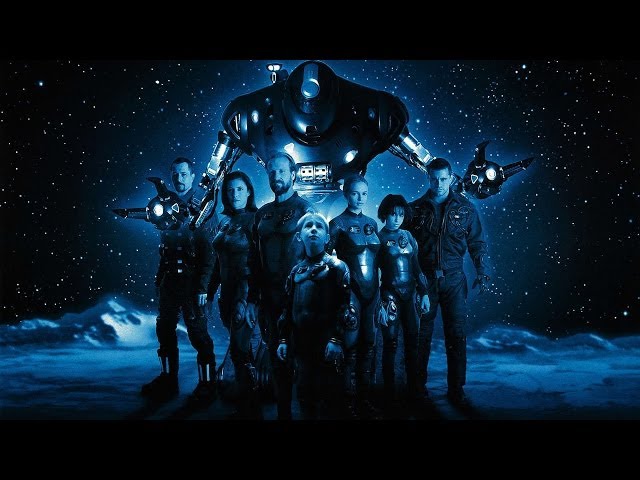The image, serving as an advertisement for a science fiction movie, features a space-themed background dominated by a stark black sky scattered with white stars and hints of a planetary surface or asteroid. At the center of the scene stands a towering robot, characterized by a shiny black body, faceless silver arms, and three-pronged claws, with its metallic hands overlapping. Surrounding the robot are seven individuals, clad in matching black bodysuits and moon boots, emphasizing their cohesive team appearance. Among them are four men and three women, showcasing a range of hairstyles and metallic suits. A notable figure is a young boy positioned at the forefront, looking upwards with a sense of concern, possibly suggestive of his role as the protagonist. The overall image maintains a bluish tint, enhancing the otherworldly atmosphere and blending the human figures and the imposing robot into the deep space aesthetic.